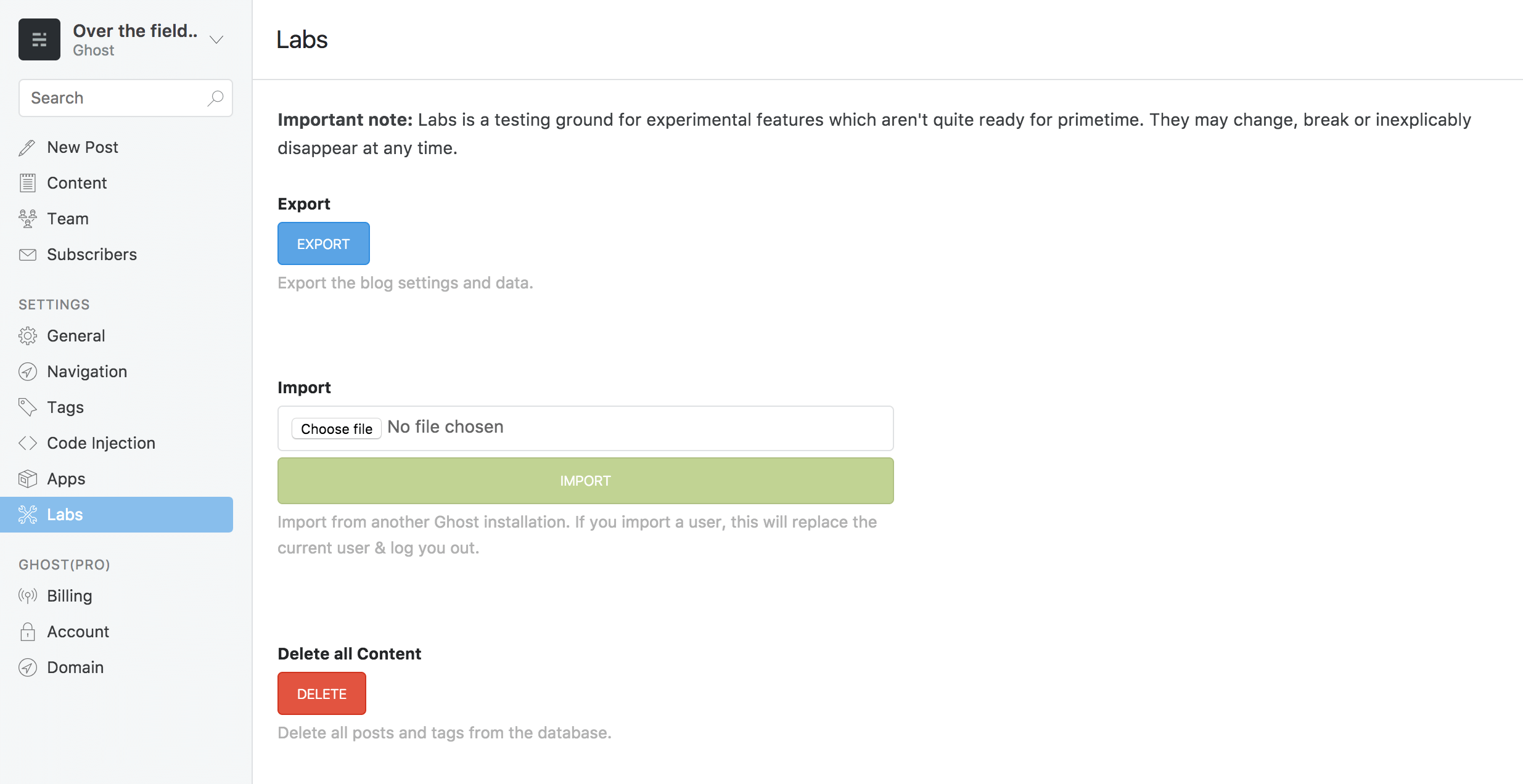A detailed view of a website's settings interface is captured. The left panel is set against a gray background and includes various navigation options listed vertically. At the top, there is a section labeled "Over the field" with "Ghost" underneath. Below this, there is a "Search" bar which is currently empty, indicated by a white box.

The navigation menu includes the following options: New Post, Contain, Team, Subscribers, Settings, General, Navigation, Tags, Code Injection, and Apps. Below these, a highlighted option in blue reads "Labs."

Further down, there are additional menu items: Ghost Pro, Billing, Account, and Domain. 

On the right side of the interface is the main section labeled "Labs." There is an important note stating, "Labs is a testing ground for experimental features which aren't quite ready for prime time. They may change, break, or inexplicably disappear at any time."

Directly below is an "Export" section with a blue button labeled "Export." The explanatory text suggests that this button allows users to export the blog settings and data.

Adjacent to the export option is an "Import" section with a "Choose file" button, indicating no file has been chosen. A green "Submit" button follows, though no data is available to submit.

A warning section titled "Import from another Ghost installation" explains that importing a user will replace the current user and log them out.

At the bottom, there's a "Delete all content" option. A red button labeled "Delete" is available, with a note underneath clarifying that this action will delete all posts and tags from the database.